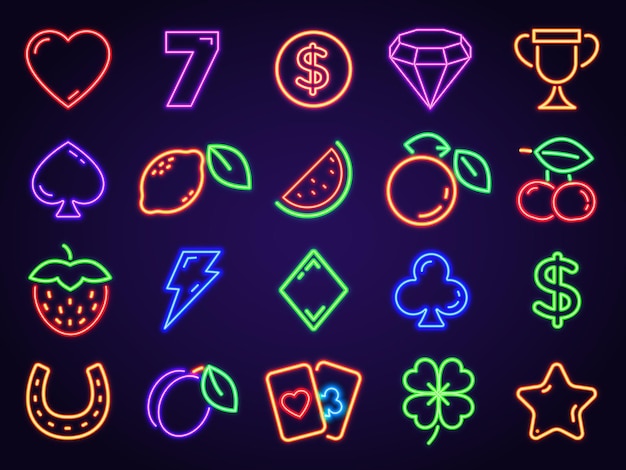This is a vibrant color photograph resembling a slot machine screen, displaying 20 brightly lit symbols organized in four rows and five columns against a purplish background. The symbols include familiar slot machine icons such as a heart, the number seven, a money sign, a diamond, a trophy, cherries, oranges, a watermelon, a lemon, a horseshoe, a strawberry, a star, a four-leaf clover, a lightning bolt, a spade, a synth symbol, and game cards. All symbols are vividly rendered in neon-like colors—red, purple, green, blue, and orange—evoking the bright and colorful energy of a Las Vegas casino. The simplistic, clipart-style design enhances the nostalgic feel, making the symbols immediately recognizable and striking.